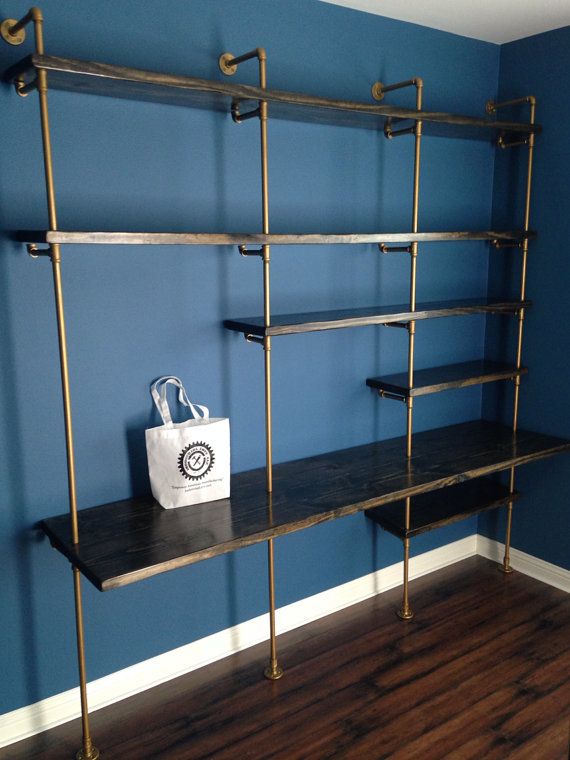In this room, a shelf unit stands against a dark blue wall, accented with a white trim. The shelving system is made of brass tubing that extends from the floor to support various shelves. There are six shelves in total, with a complex arrangement: three larger shelves spanning all four brass pipes—two at the top and one at the bottom—and three smaller shelves supported by just three pipes. The dark cherry wood floor, possibly tiled with a high gloss, adds a touch of elegance to the space. The only item on the shelves is a white canvas bag with straps and a logo that resembles a Rotarian symbol—a gear with what looks like a hammer and a saw—though the text is too small to read.